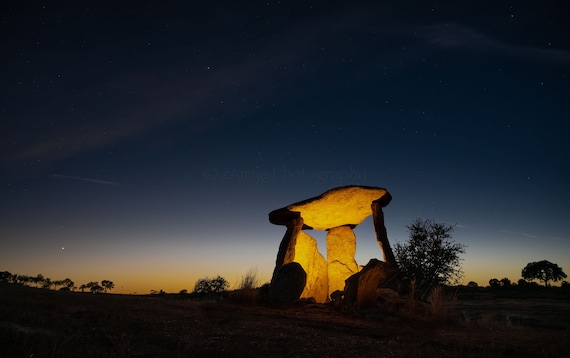The photograph captures a desolate, open landscape at dusk, with the last traces of sunlight painting the horizon in hues of gold, orange, and purple. The night sky has taken on a deep navy blue color, transitioning to darkness as you move upward from the horizon. Rolling hills and sparse grasslands are visible, dotted with occasional distant trees. The central focus of the image is a primitive, man-made stone structure reminiscent of Stonehenge. This consists of several large slabs of stone arranged to form a rudimentary shelter or gazebo-like figure, with a flat, jagged rock positioned horizontally on top, supported by three vertical pillar stones. The structure is internally illuminated, possibly by fire or another light source, casting a warm yellow glow that contrasts strikingly with the encroaching night. This light highlights the texture and form of the stones, making the structure stand out vividly against the dim landscape. The mysterious and serene scene suggests a remote location, possibly a grassland or desert, underlining the timeless and enigmatic quality of the stone structure.